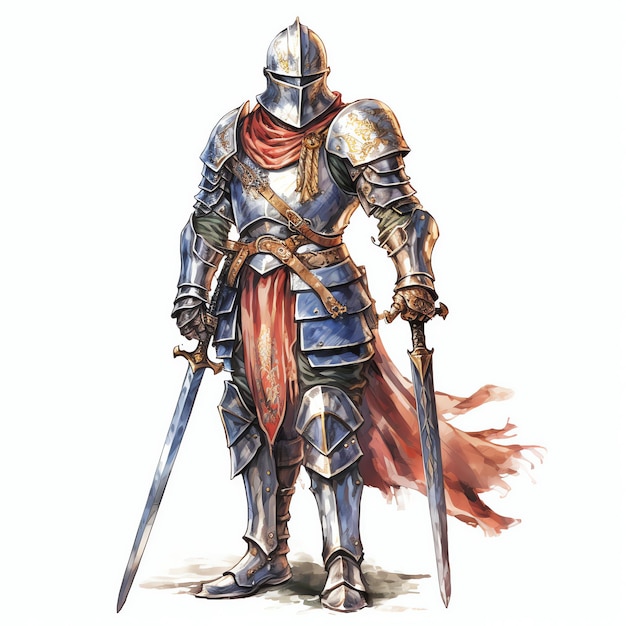The image depicts an intricately detailed painting or drawing of a soldier clad in medieval Roman-inspired armor. The figure is encased in silver-tinted metal armor from head to toe, including a fully enclosed helmet with a narrow slit for the eyes. The armor features large shoulder pads, a chest plate, and thick, ornate knee guards, and metal shoes. The soldier is adorned with a reddish-orange tunic around the neck, complemented by a red sash or cloth that extends from the waist and flows behind, resembling a cape billowing in the wind. The figure is also equipped with two swords, one in each hand, with shiny silver blades and brass or bronze handles, both tips pointed downward towards a visible gray-black patch of ground. The overall color palette includes hues of blue and gold, adding to the regal appearance of the warrior in this striking, background-free composition.